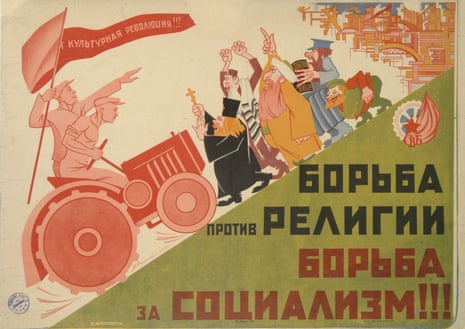This image depicts a Russian propaganda poster characterized by its striking and vivid elements. Dominating the scene are two workers aboard a vibrant orange and pink tractor, positioned diagonally from the lower left-hand corner, climbing a steep gradient towards the upper right-hand side. The workers are holding a banner inscribed with Russian text. Facing the oncoming tractor, a group of civilians, including bishops, priests holding crosses, and a bearded Muslim man with a white hat, stand with arms raised in protest. The religious figures, clad in varying traditional garments, appear to be attempting to halt the tractor's progress. The poster features a notable green triangle at the bottom right, symbolizing a hill, adorned with Russian text in black and red letters, with the red portion followed by three exclamation points. The upper right-hand corner contains an indistinct emblem, adding to the propaganda motif. In the background, several buildings can be seen, providing context to the dramatic confrontation.